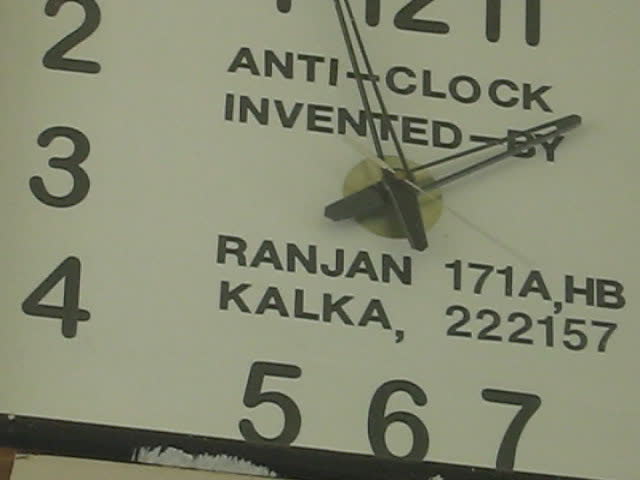This image showcases a large, uniquely designed clock face known as the "Anti-Clock." The clock face features sizable numbers arranged in a counter-clockwise direction, with 12 at the top and 6 at the bottom. Unlike traditional clocks, the numbers 1 through 12 progress counter-clockwise from the top right around to the top left. Below the clock hands, there is an inscription that reads "Anti-Clock Invented by Ranjan Kalka." Adjacent to this, there are additional markings, "171A, HB," followed by another sequence, "222157." The overall design emphasizes the anti-clockwise progression of time, distinguishing it from conventional clocks.